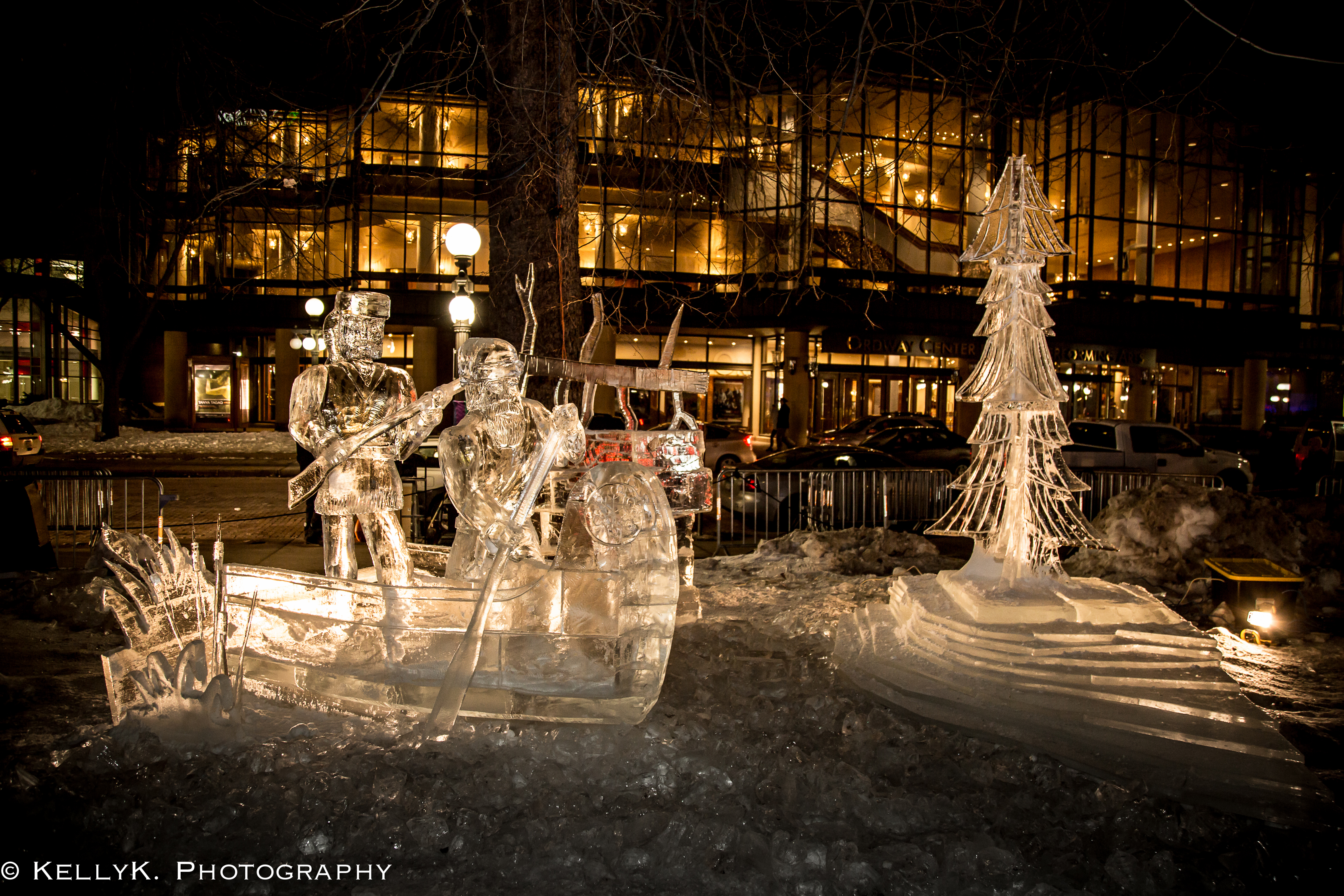This nighttime photograph captures a stunning outdoor ice sculpture display, likely taken in a city park setting. At the center, silhouetted against a brightly illuminated building, two detailed ice sculptures dominate the scene. On the left, a canoe-carved from ice holds two explorers; the one at the back stands poised with a musket, reminiscent of a frontiersman, while the figure at the front kneels, seemingly paddling through the intricately sculpted waves of ice. Interestingly, the front figure has a semblance to Santa Claus, possibly hinting at a festive theme. To the right of the canoe, a tall, narrow ice sculpture resembling a Christmas tree stands atop a striated ice platform, adding to the wintry ambiance. The entire scene, from the illuminated backdrop to the meticulously detailed ice sculptures, exudes a magical, festive atmosphere, suggesting a celebration like an Ice Festival. The photograph bears a signature in the lower left, attributing the work to Kelly K Photography.